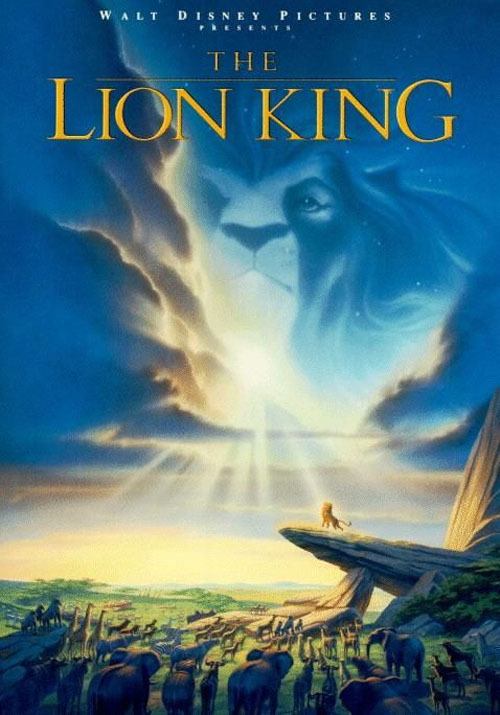This is a highly detailed movie poster for Walt Disney's 1990s animated classic, "The Lion King." At the very top center of the poster, in white letters, it reads "Walt Disney Pictures presents," followed by the movie title in large yellow text: "The Lion King." The background features a beautifully painted sky with varying shades of light and dark blue, with clouds parting to reveal a semi-transparent lion's face. The sun's rays beam down dramatically onto Pride Rock, a prominent rock formation jutting upward at a slight angle. Standing atop Pride Rock is a lion, presumably Simba, gazing upwards. Below, a variety of African animals, including elephants, giraffes, and possibly gorillas, are depicted surrounding the rock formation. The overall image captures the essence of the movie's awe-inspiring landscapes and its central theme of the animal kingdom.